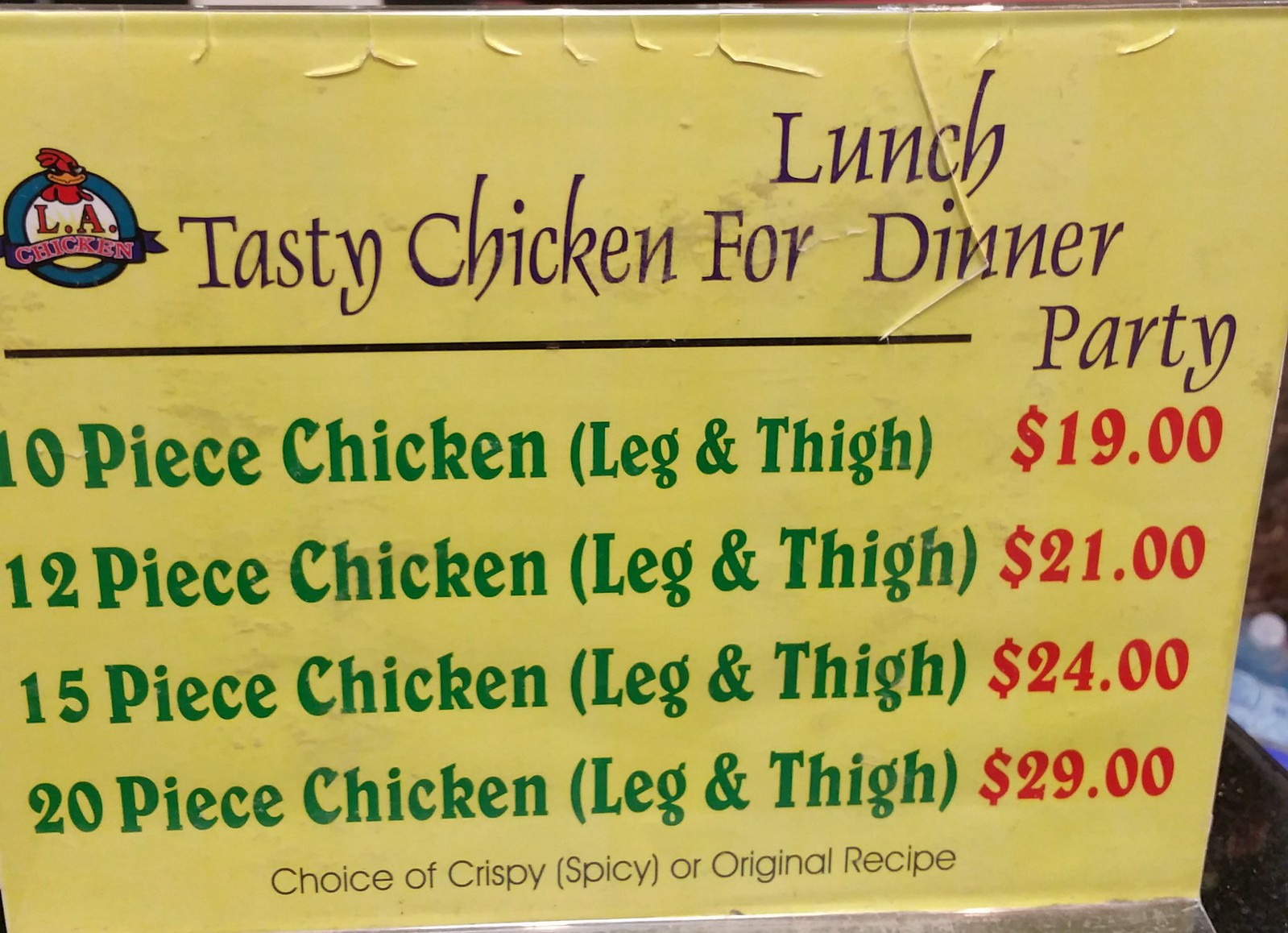An aged and weathered outdoor sign advertises "LA Chicken." The sign's once vibrant yellow paint is peeling, revealing the elements' impact over time. This battered facade is encased in a broken plexiglass shield, offering a glimpse into its former, more pristine state. In the top left corner, a small blue section adds a contrasting hue. At the sign's top, a whimsical red cartoon rooster stands proudly, symbolizing the brand. Below the rooster, bold text proclaims: "Tasty chicken for lunch, dinner, and party." A horizontal line divides the header from the menu beneath, listing options in green text with prices highlighted in red. The menu offers various quantities of chicken legs and thighs: 10 pieces for $19, 12 pieces for $21, 15 pieces for $24, and 20 pieces for $29. Under the menu, a note informs customers of their choice of preparation: "crispy (spicy or original recipe)."